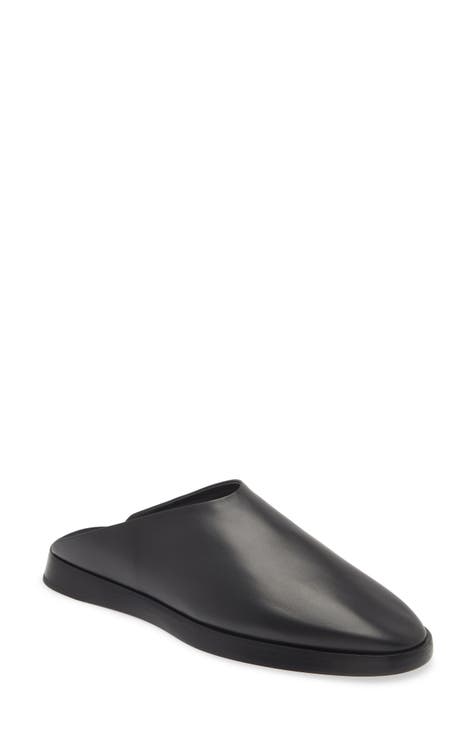The image showcases a single black slip-on shoe, prominently displaying the top and right side. Crafted from shiny black leather, the shoe catches ambient light, highlighting its sleek appearance. It features a flat, inch-thick black sole, characterized by its casual but polished style. Positioned with the toes pointing towards the bottom right and the heel towards the left, the sandal extends further back than typical styles, almost reaching the ankle, with an open back. The background is a clean, unobtrusive white, providing no border or additional context, ensuring the focus remains solely on the shoe.